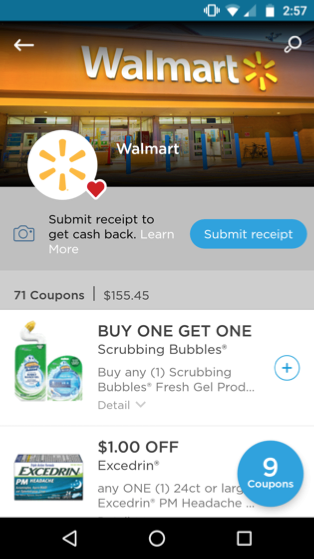This is a detailed screenshot of the Walmart app interface. At the top, there is a teal status bar displaying the time at 2:57 on the right side, alongside icons indicating the battery level and phone vibration status. Below this status bar, there is a header featuring a picture of a Walmart store along with the Walmart logo adorned with a red heart. 

In this header section, there is a prominent blue "Submit Receipt" button, accompanied by a text prompt to the left that reads "Submit Receipt to get cash back." At the very bottom of this header section, there are details noting "71 coupons" and "$155.45."

Beneath the header, the screen transitions to a white background displaying two product items. The first item listed is Scrubbing Bubbles, offered on a "buy one get one free" promotion for any Scrubbing Bubbles Fresh Gel product. There is a blue plus sign to the right of the product name. The second item is Excedrin, featuring a discount of $1 off and a blue circle indicating "9 coupons."

The bottom of the screenshot includes a black stripe, which is part of the phone's hardware interface and not the app itself.